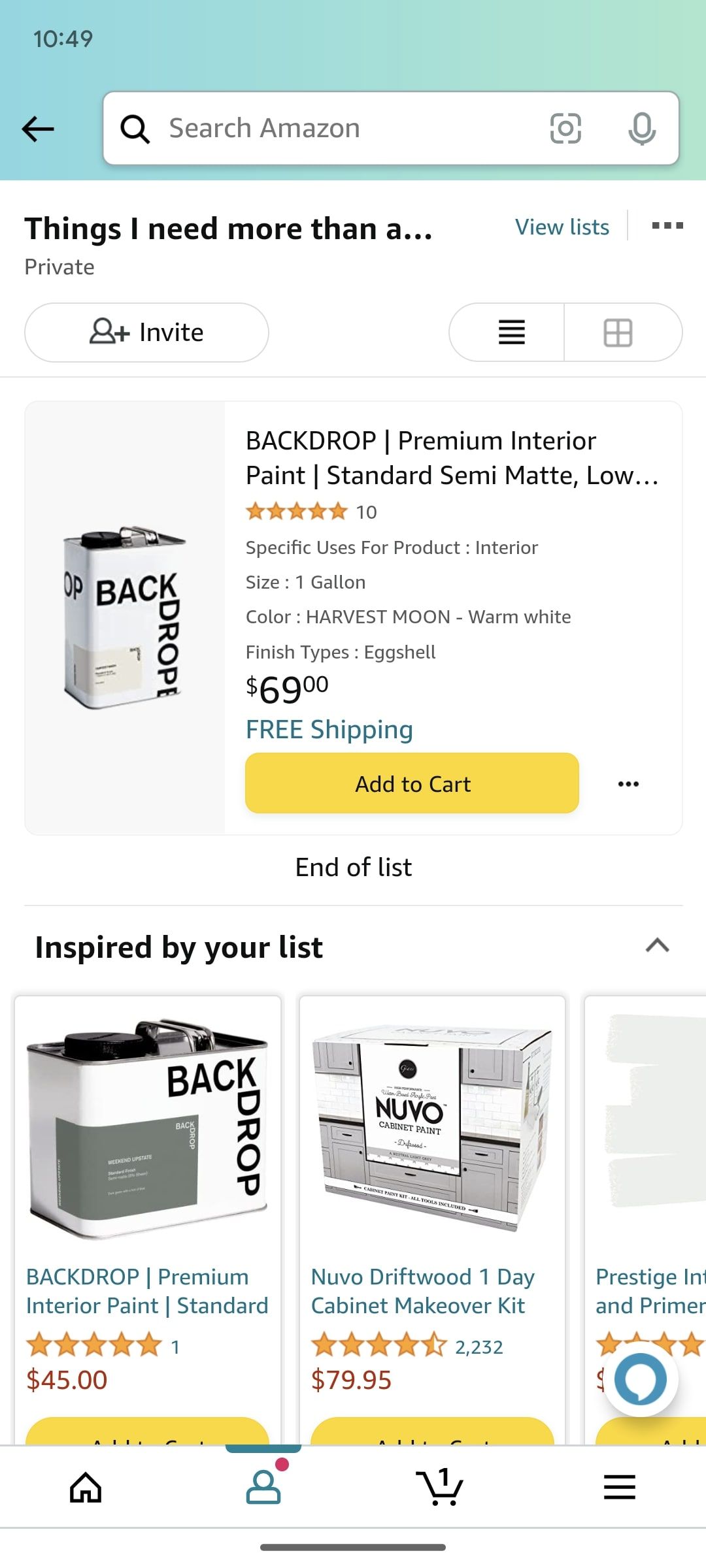**Caption:**

The image showcases an Amazon profile with a private list titled "Things I Need More Than Anything." At the top of the screen, there's a search bar with the text "Search Amazon." Below the list title, options to "View List" and a "Private" label are visible, accompanied by an "Invite" button. The menu icon is situated to the right.

The primary item in the list is a "Backdrop Premium Interior Paint," described as follows:
- Type: Standard Semi-Matte, Eggshell Finish
- Specific Use: Interior
- Size: One Gallon
- Color: Harvest Moon Warm White
- Price: $69 per gallon
- Option: Add to Cart

The section ends with "End of List." Directly below, there's a segment titled "Inspired by Your List," featuring additional products:
- Premium Interior Paint at $45
- Nuvo Driftwood 1-Day Cabinet Makeover Kit at $79

Towards the bottom, a profile picture with a house icon is depicted, next to several menu options including "Messages," "Cart (1 item)," and menu bars.